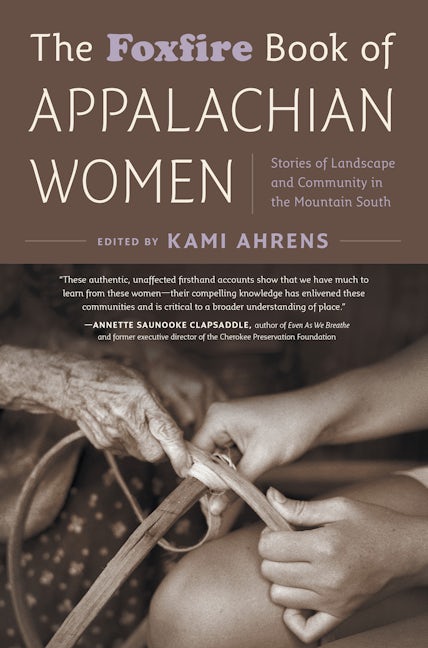The cover of "The Foxfire Book of Appalachian Women: Stories of Landscape and Community in the Mountain South," edited by Kami Ahrens, is a powerful visual and textual blend that highlights the wisdom and contributions of Appalachian women. The top half of the cover features the book’s title in white and light purple text against a brown background, with the word "Foxfire" standing out in a unique font. Beneath the title, a quote by Annette Saunooke Clapsaddle, author of "Even As We Breathe" and former Executive Director of the Cherokee Preservation Foundation, underscores the importance of these authentic, first-hand accounts, emphasizing the critical role these women’s knowledge plays in understanding community and place.

The lower half of the cover showcases a poignant black-and-white photograph. An elderly hand on the left holds a thick, pliable piece of wood, which is being passed to younger hands on the right, indicating the transmission of traditional skills. The image suggests a possible weaving or binding process, symbolizing the intergenerational transfer of knowledge. The earthy tones and focused composition of the image complement the book’s theme of enduring community and tradition in the Appalachian region.